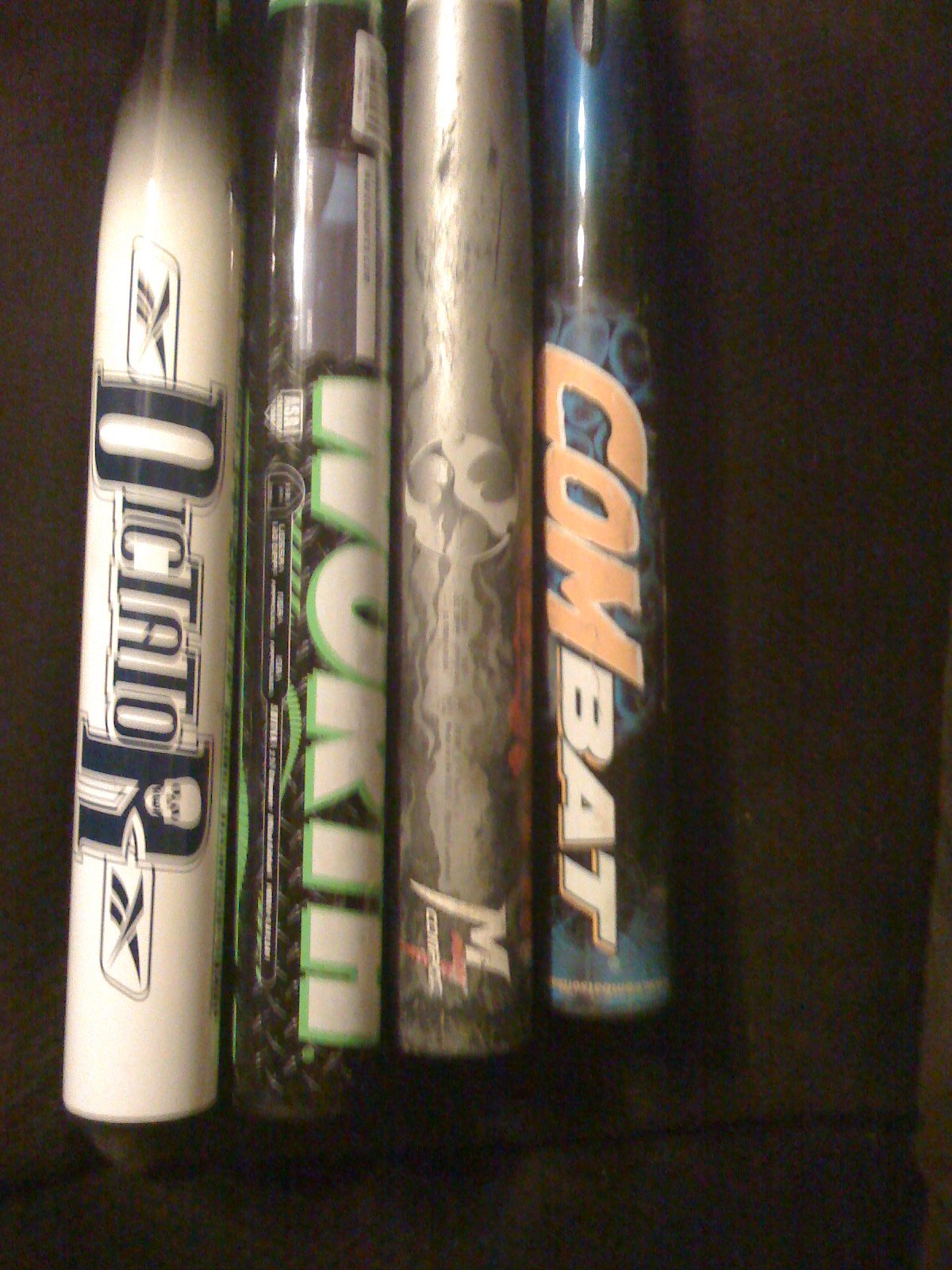This image is a close-up photograph of the barrels of four aluminum baseball bats lined up side by side against a solid black background. The bats, which are not typical of professional leagues, reveal distinct styles, colors, and branding. Starting from the left, the first bat is white with navy blue lettering that reads "Dictator"; the 'R' includes a skull motif and the bat features Reebok logos. The second bat is predominantly black with partially visible white text outlined in neon green, likely reading "Woken." The third bat has a metallic silver finish with a blurry white decal, possibly showing a face with sunglasses and an 'M' letter. The final bat stands out with its blue body and bold "Combat" branding; 'Com' is displayed in orange letters, while 'Bat' is in white, all set against the dark background.